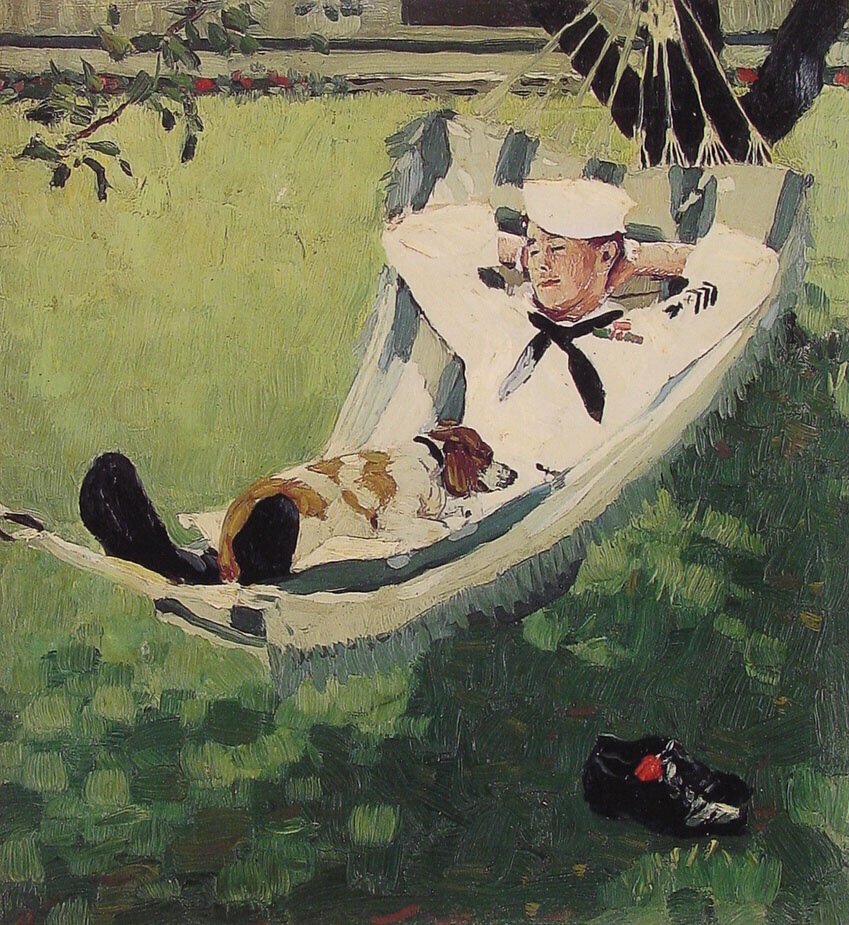This watercolor painting depicts a serene outdoor scene of a sailor taking a nap in a hammock. The sailor, clad in a white uniform adorned with three stripes on the sleeve and a black necktie, has removed his black shoes, which rest on the grass beneath him. His eyes are closed, and he has his hands behind his head, relaxing in the hammock. A brown and white dog, resembling a beagle, lies peacefully on his lap. The hammock is strung between the branches of a tree, which are visible to the left, and stretches over a lawn mottled with dark and light green grass. In the background, a small portion of a house and the suggestion of a fence or possibly a wagon wheel can be seen, enhancing the idyllic, restful atmosphere of the scene.